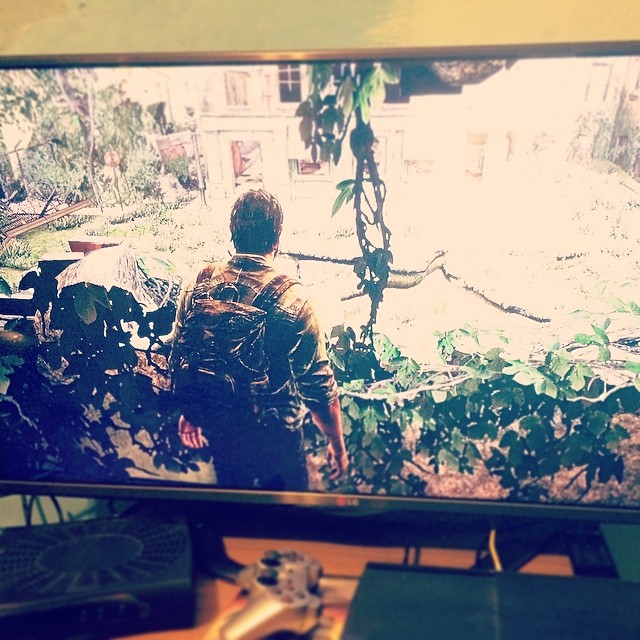The image depicts a flat-screen television with a black border sitting on a brown stand, emblazoned with an LG logo on its bottom edge. The wall behind the television is green and white, and there are distinct lines extending from behind the TV, possibly cables. In front of the screen, on the stand, lie two books and a silver video game controller with black analog sticks. The television displays a scene from a video game, featuring a man standing in a lush, greenery-filled yard with hanging vines, facing a partially visible white house bathed in bright sunlight. The house has a glass-door entry and an outdoor light situated to the left of the door. Additionally, a remote control is noted amongst the small electronics on the stand. The setting suggests a casual, lived-in room, potentially a living room or a personal study area.